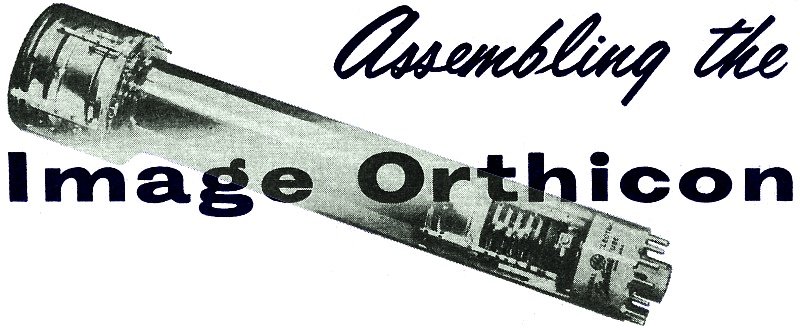The image appears to be a logo or header featuring the title "Assembling The Image Orthicon." The phrase is written in two different fonts: "Assembling The" is in a cursive script, while "Image Orthicon" is in a bold, black print font. The background showcases a stylized grayscale scan of an apparatus, likely the Image Orthicon itself, which looks similar to a flashlight or a lightsaber handle from Star Wars. This machinery has a rounded end, a thinner cylinder-like handle, and a bottom section that appears capable of screwing or plugging into a fixture, featuring some pins and silver ridges. The device looks worn and used, and there is a faint, small inscription at the bottom, though only the letter "L" is legible. The overall color scheme of the background object is shades of gray with distinct black accents.